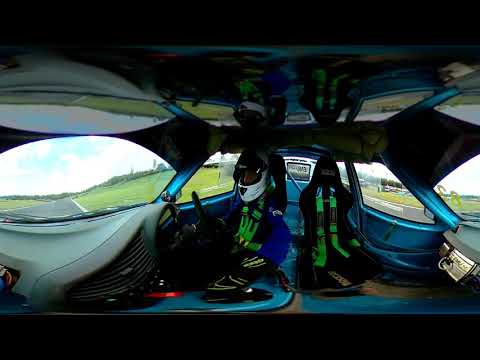The image depicts the interior of a racing car, captured from a dashboard-mounted camera with a fisheye filter effect causing a curved, distorted view. The racing car features two black seats equipped with green racing harness seat belts. The left seat is occupied by the driver, who is dressed in a blue jacket and wearing a white and black helmet, gripping the steering wheel. The right seat remains empty. Visible through the windows is a gray track bordered by lush, green grass, set beneath a blue sky dotted with white clouds. The vehicle's interior is primarily blue, and there are glimpses of equipment hanging from the ceiling, possibly shoes or other racing-related gear. The image also includes horizontal black strips at the top and bottom, underscoring the unique perspective of this dynamic, action-filled scene.